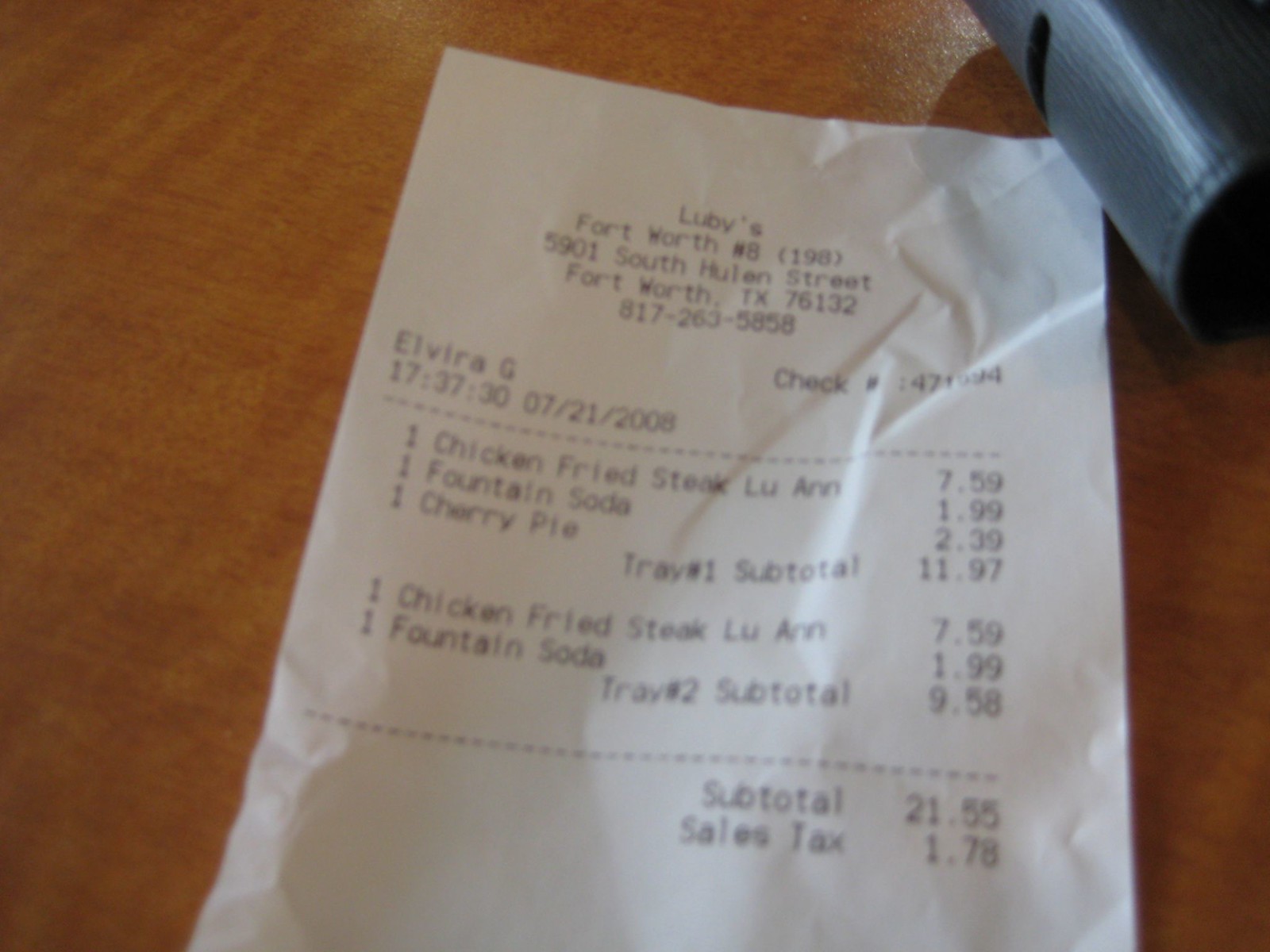In this indoor color photograph, a wooden table hosts a slightly wrinkled, white receipt with black lettering. The receipt is from Luby's at Fort Worth, location number 8198, situated at 5901 South Hulen Street, Fort Worth, Texas 76132, with the contact number 817-263-5858. The transaction, handled by the server Elvira G., occurred on July 21, 2008, at 17:37:30, under check number 47194. Listed items include a Chicken Fried Steak Luan for $7.59, a Fountain Soda for $1.99, and a Cherry Pie for $2.39, amassing a tray 1 subtotal of $11.97. In addition, another Chicken Fried Steak Luan and Fountain Soda make up tray 2's subtotal of $9.58. Together, these subtotals combine to $21.55, with an added sales tax of $1.78. Also visible in the image, next to the receipt, is the edge of a black leather portfolio.